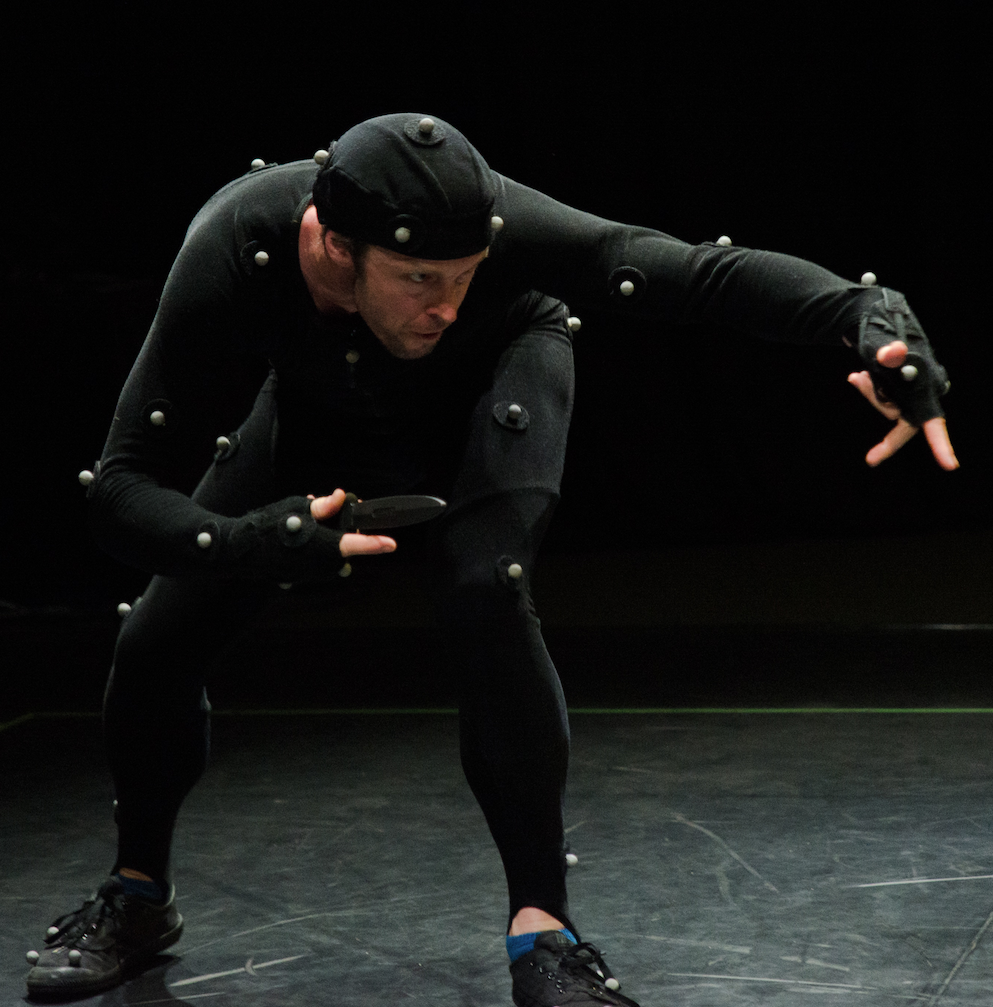The image depicts a man wearing a full-body motion capture (mocap) suit, which is entirely black, including a tight shirt, tights, cap, and shoes, with only his face and fingertips exposed. The suit is adorned with several small, deep grey tracking markers positioned at joint areas to capture and translate his movements for digital animation. The man, who appears to be portraying a character for a movie, show, or video game, is bent at the waist in a dynamic pose, with his head near his groin. His left arm is extended outward and pointed downward, while his right arm is closer to his body, holding a small black knife. His face shows a grimace, indicative of effort, suggesting he might be playing a villain. There is no visible background, implying he is performing in front of a green screen.